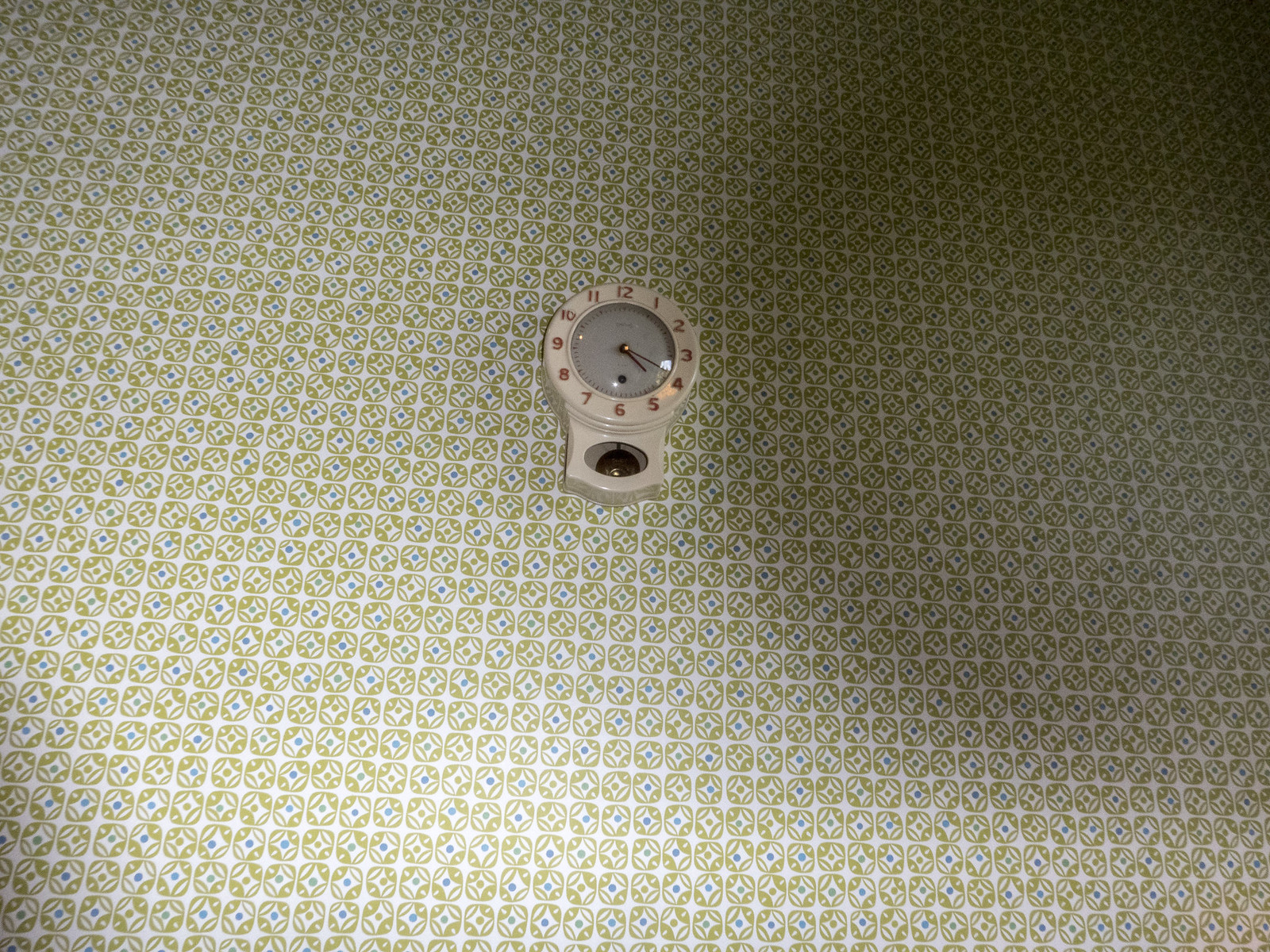The image features a wall adorned with wallpaper characterized by a predominantly white background interspersed with soft-edged, green squares. Each green square contains a central white shape that houses a small blue dot, creating a pattern that extends across the wall. At the center of the image, a round clock is mounted on the wall. This clock appears to be made from a reflective material, possibly tin or porcelain, with a beige outer casing. The face of the clock is white and protected by a glass cover. Uniquely, the numbers are positioned on the outer rim of the reflective material rather than directly on the glass. Below the clock’s face, an oval section features a sizable gold pendulum, adding a touch of elegance to the overall design.